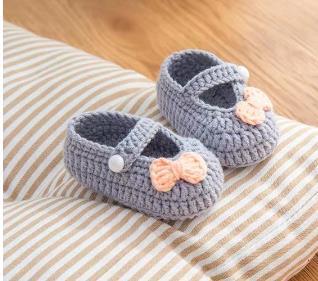The image is a close-up, square photograph featuring a pair of medium-grey knitted baby booties, adorned with delicate peach bows on each toe. The booties, secured with light blue straps fastened by round, pearlescent white buttons, are carefully positioned on a pillow or cushion with brown and white stripes. The pillow extends beyond the frame on the left, bottom right, and bottom edges of the image. The backdrop is a rich, brown wood laminate floor, emphasizing the cozy and quaint aesthetic. The composition centers on the booties and pillow, devoid of any other objects or people, highlighting the charm and intricate details of the handcrafted footwear.